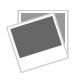This detailed artistic sketch features a vibrant red parrot perched on a semi-mossy tree branch. The bird stands out against an off-white background, facing right with its tail fanned towards the lower left corner. Its striking plumage showcases blue feathers interspersed with red on its wings and tail, with a lighter blue hue tipping the tail feathers. The parrot's cheeks and an area under its eye are highlighted with a bright blue, contrasting with its dark and light brown beady eye. The beak is a mix of gray and peach, with a hint of gold at the tips. The bird grips the branch with its brown talons, which are detailed with some missing bark and a cut end, and hints of green moss. Below the parrot, a cursive inscription reads "La Perruche large queue PL78", followed by additional, less legible text. The illustration's meticulous details suggest it could be a vintage book's illustration, capturing the parrot’s vivid colors and intricate beauty.